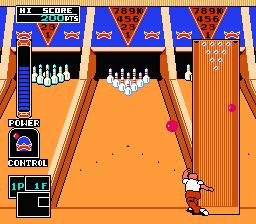The image captures a small square frame from a bowling video game, focusing on the central lane with partial views of adjacent lanes. Dominating the scene, a red triangle with black numbers and a blue border adorns the wall above the pins, providing a visual focal point for players. The pins, arranged in their starting positions, each feature a distinctive red stripe around their necks. In the bottom right corner, a player clad in a white shirt and red pants is captured mid-action, having just released the bowling ball. The ball appears to be halfway down the lane, precariously veering towards the right gutter.